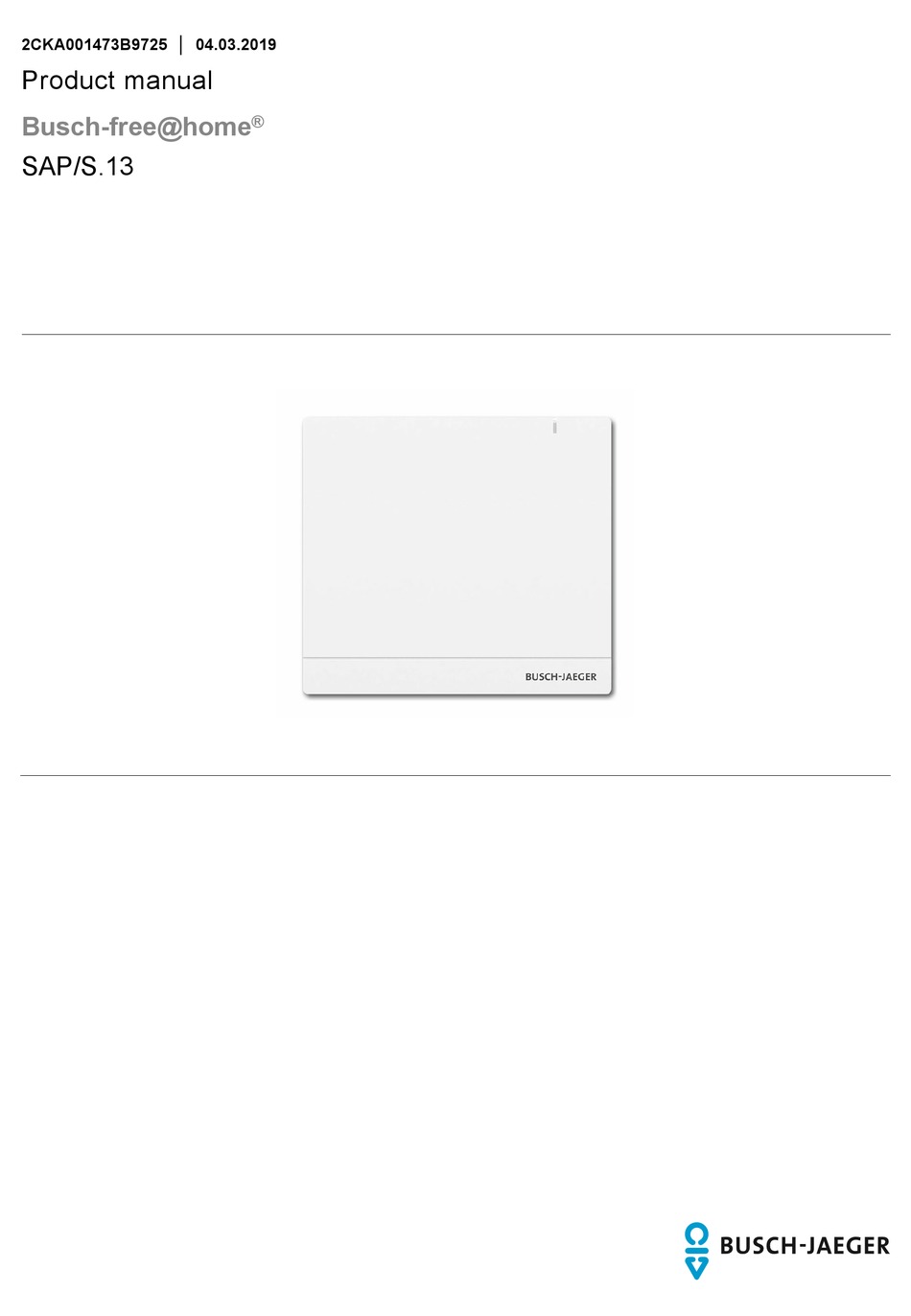This is a screenshot from the Busch-Jaeger website. The name "Busch-Jaeger" is spelled B-U-S-C-H J-A-E-G-E-R. The screenshot features an icon resembling a semi-circle with a bar and a triangle beneath it. The user has purchased a product manual with the school number 2CKA00147-3B9725. The date on the screenshot is April 3rd, 2019. The product is labeled as "Bush-free@home® SAP/S.13." Additionally, there are two lines within the image, between which there is an image of a Busch-Jaeger product, possibly a modem or a laptop. The product is square-shaped with a line at the bottom displaying the Busch-Jaeger name. The context suggests this might be an examination of the website and its features.